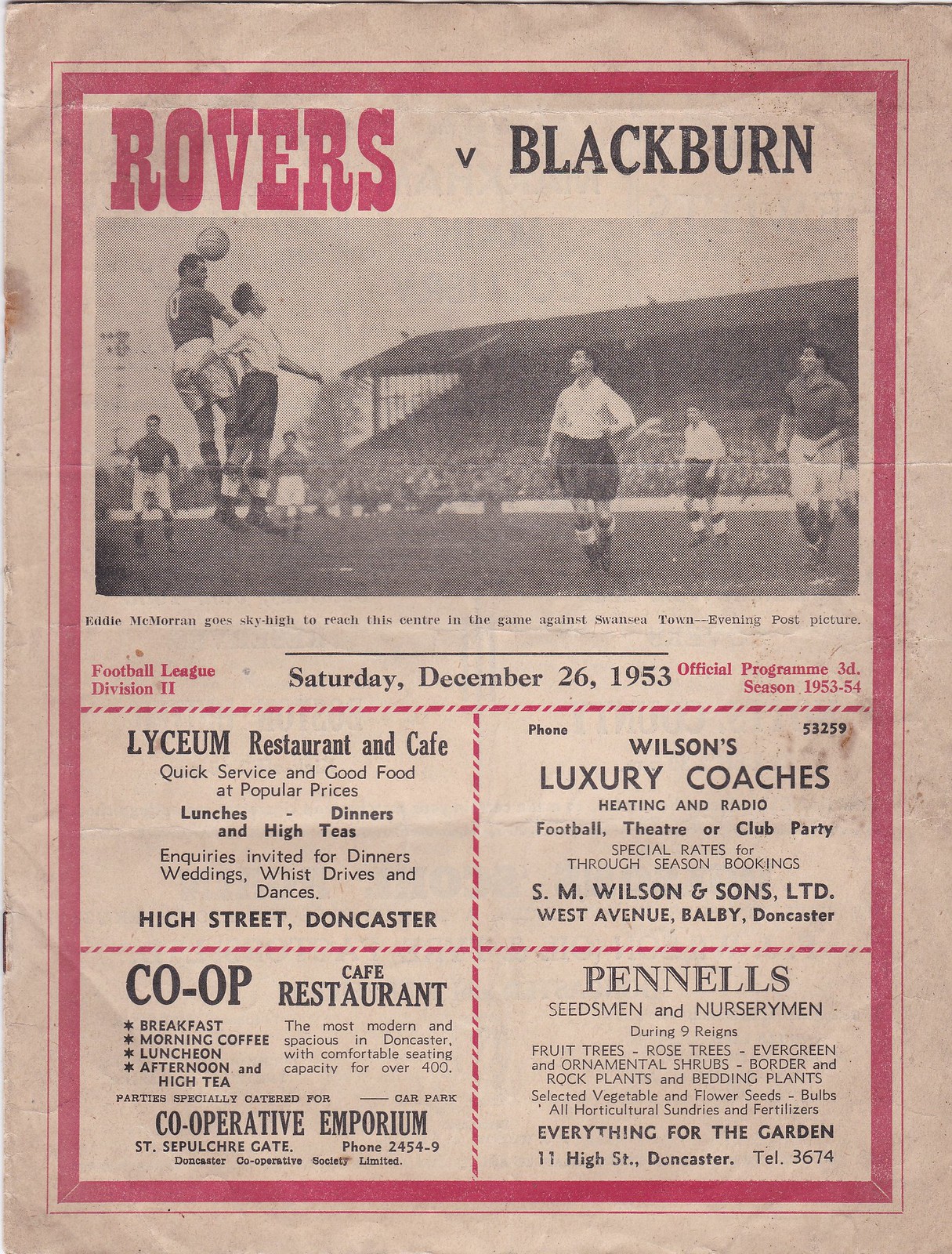The image features a single, prominently centered, vintage football program, set against an aged, tannish sheet of paper. The program, which has yellowed over time, boasts a striking red border with predominantly black text accentuated by red highlights. At the top, in bold red letters, it reads "Rovers vs. Blackburn," signaling a historic match held on Saturday, December 26, 1953, during the Football League Division 2 season of 1953-54. Below this title, there's a dynamic black-and-white photograph of football players in action within a stadium; two players are seen leaping to head the ball, capturing a moment of intense competition. The text further emphasizes Eddie McMorrin’s sky-high reach in a game against Swanson Town. The lower portion of the program features advertisements for local businesses, including the Lyceum Restaurant Cafe, Wilson's Luxury Coaches, Peno's, Co-op Cafe Restaurant, and Pennell's Seedsmen and Nurserymen. This official program appears designed for spectators attending the game, providing a snapshot of mid-20th-century football culture.